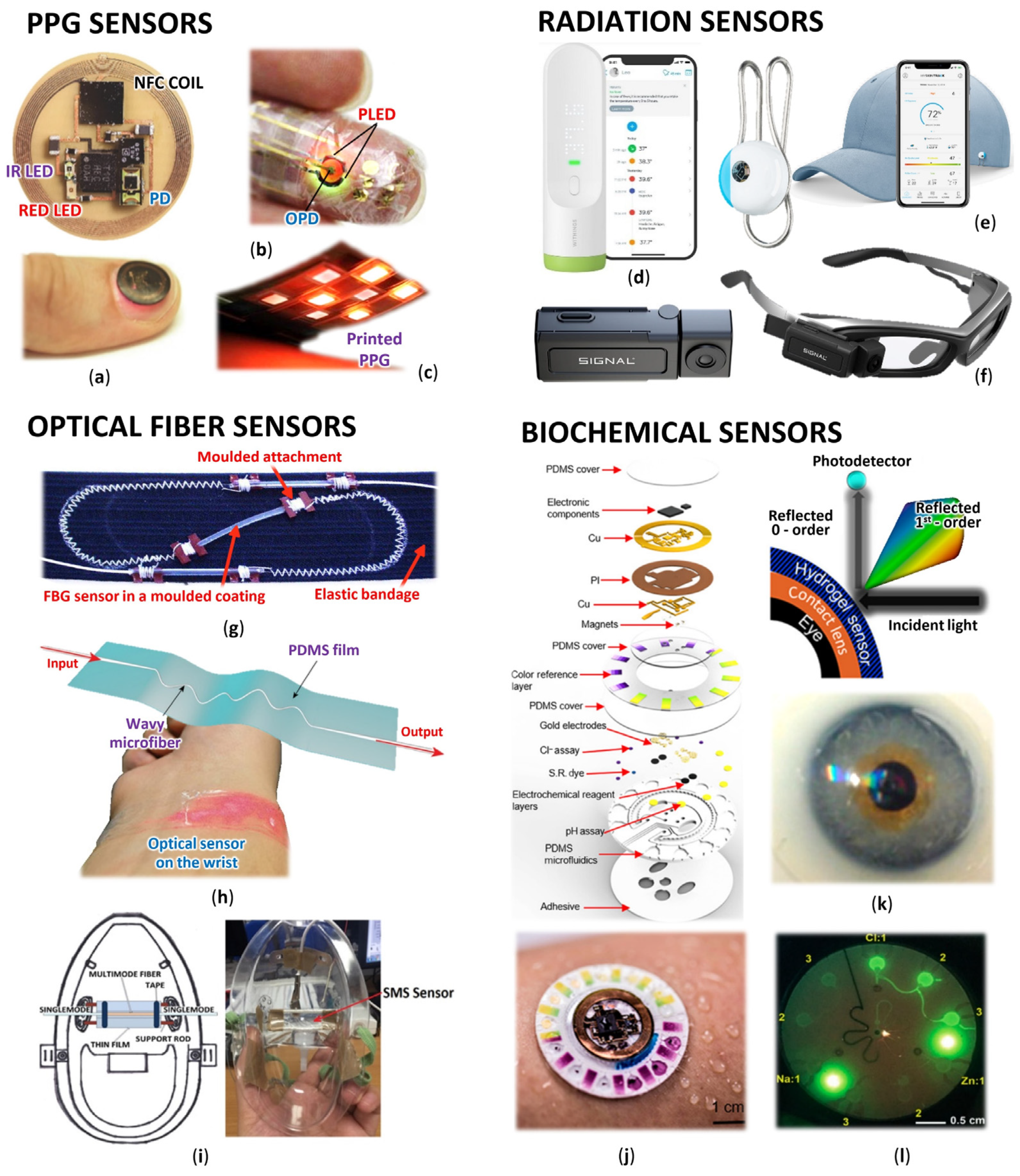The image is a detailed collage of various types of sensors, divided into four main categories, each represented in its own section. In the upper left quadrant, labeled "PPG Sensors," there are illustrations of printed PPG sensors applied to fingers, with sub-labels A, B, and C highlighting different views and components, including little red lights. The upper right quadrant, titled "Radiation Sensors," features several depictions including a smartphone with an attached sensor, glasses with an integrated sensor, and another sensor resembling a kid's toy, all marked with labels D, E, and F. In the lower left section, "Optical Fiber Sensors," includes imagery such as a sensor wrapped around a hand, and a cranium-shaped device labeled as an SMS sensor, with sub-labels G, H, and I. The lower right section, titled "Biochemical Sensors," displays the detailed breakdown of sensor components, an image of the sensor on wet skin, a photodetector, an eyeball, and a green orb-like structure, labeled with J, K, and L. Each section is accompanied by detailed images and labels, making the collage an intricate and informative guide on various sensor types.